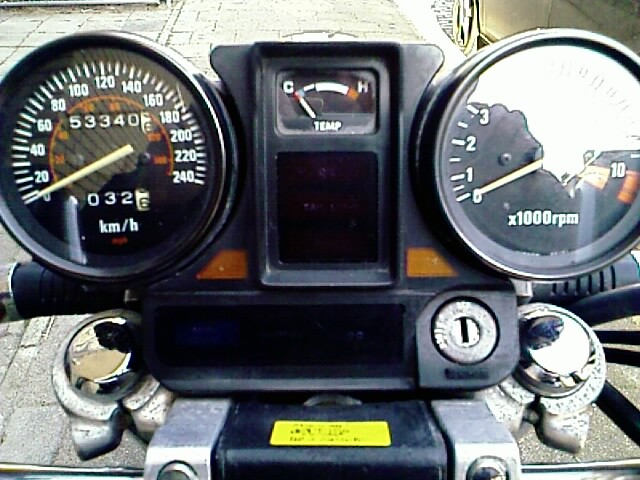This detailed caption provides a vivid description of the image:

"The photograph presents a rider's perspective from the front of a motorcycle. Dominating the foreground are the instrument dials: a round speedometer on the left marked in white numbers and strokes against a black background, measuring speeds from 0 to 240 kilometers per hour. It features an inner ring highlighted in orange. To the right of the speedometer is the tachometer, monitoring the engine's rotations per minute, and centrally positioned above them is the temperature gauge, labeled 'TEMP' with a 'C' for cold on the left and an 'H' for hot on the right. The black handlebars, accented with silver circles, frame the instruments, with the silver keyhole visible just below the gauges. The scene is set on a gray cobblestone surface, suggesting a driveway or sidewalk, with a white car partially visible in the upper right corner. This contextual detail supports the impression that the motorcycle is parked in a residential area."